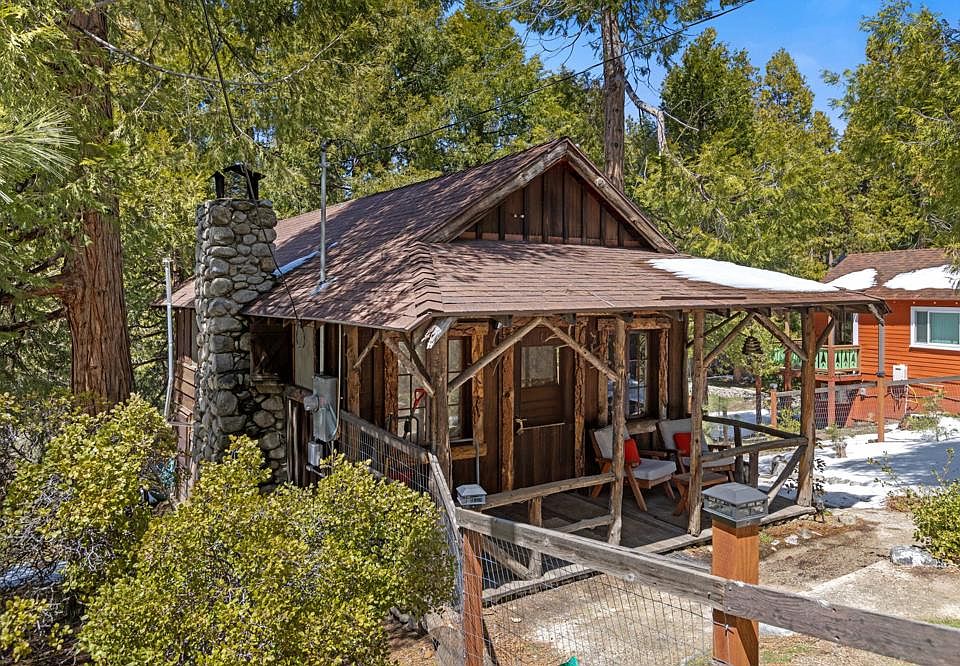The image depicts a serene outdoor scene featuring two rustic cabins nestled amidst a forest of tall, green trees under a blue sky. The primary cabin in the foreground is a dark brown wooden structure with a distinctive stone chimney on its left side. It has a cozy front porch equipped with two wooden chairs adorned with red throw pillows and off-white cushions. The cabin's design includes brown wooden railings, trim around the windows and door, and a brown roof that matches the rest of the structure. A wire and wood fence with cap-topped posts encircles the property, blending into the scenic environment.

In front of the cabin, the ground appears to be covered with beige dirt, possibly mingled with patches of melting snow. Various plants and bushes surround the area, adding to the rustic appeal. In the background, another cabin, painted an orangish-brown color, stands partially visible to the right. This second cabin features a green balcony and similarly has patches of snow melting on its rooftop. The overall impression is one of peacefulness and rustic charm, capturing the essence of woodland living.